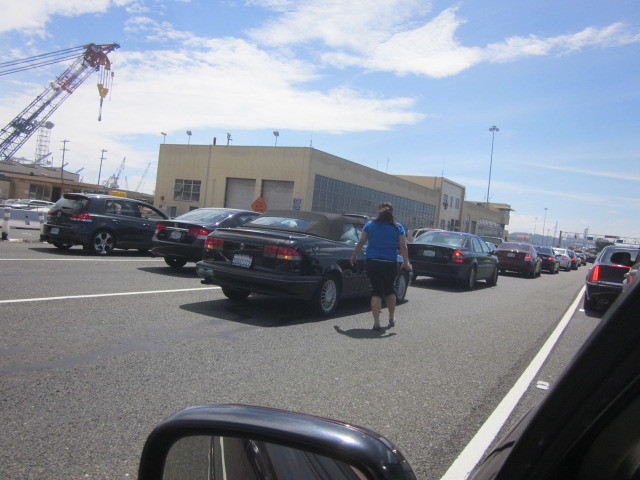The photograph, taken from inside a moving dark blue car, captures a bustling four-lane highway in an industrial area under a light blue sky with scattered white clouds. The viewer's perspective includes the partially visible side mirror in the lower right corner. Outside the open window, a tan, one-story building occupies the middle ground, with several cranes—one prominently dark blue and red with a yellow crane portion—rising to the left of it. A large parking lot filled with vehicles stretches beside the road. Dominating the center of the image is a woman with long, dark hair secured in a ponytail, wearing black below-the-knee pants, a blue t-shirt, and white shoes. She walks with her arms slightly outstretched towards a black car amidst the traffic, which includes several black cars, a maroon car, and a white car extending into the distance. The scene suggests a bright, sunny day, with some overcast areas visible on the left side of the sky.